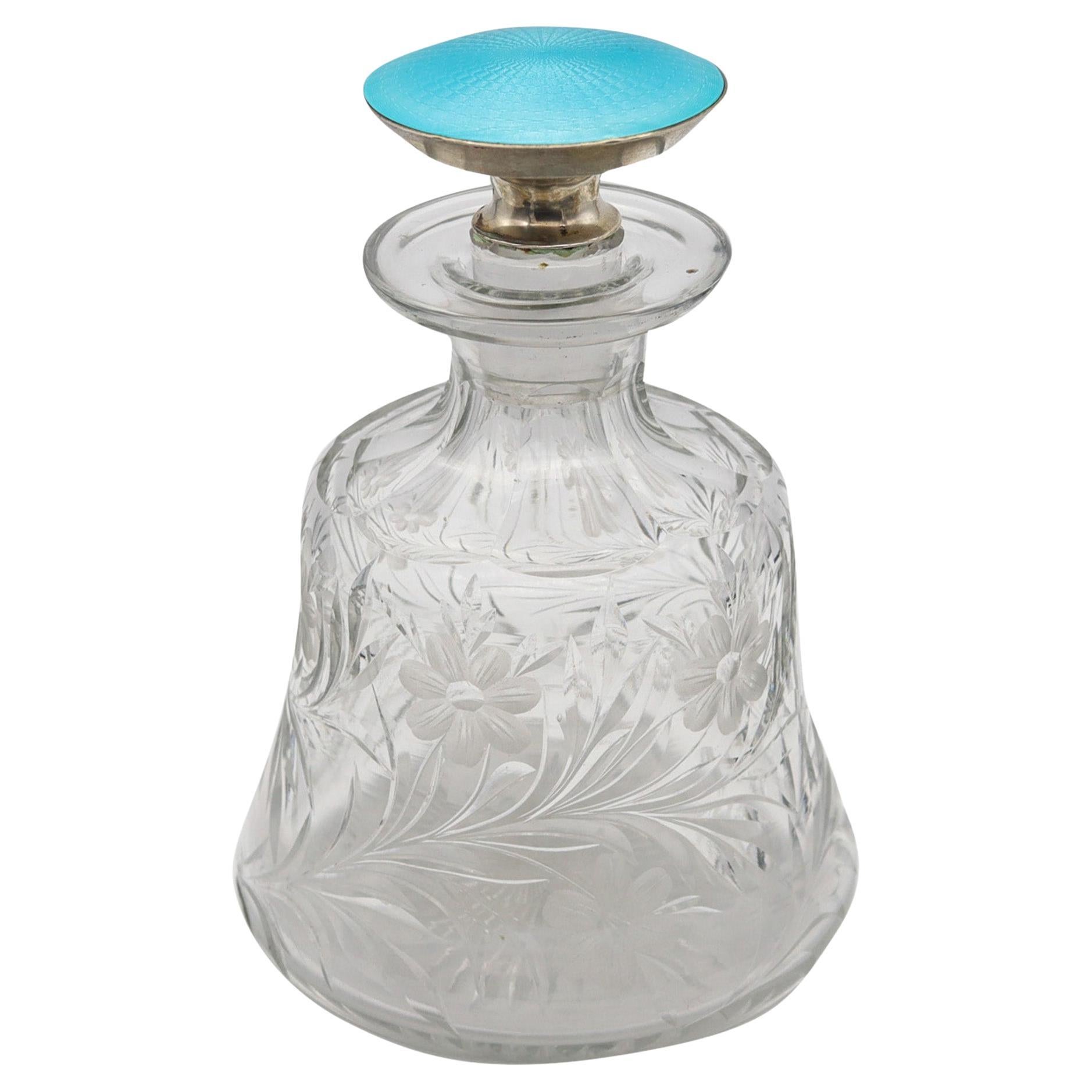The image is a color photograph in portrait orientation, featuring a glass container with a round, aqua blue lid that resembles a gem or dome shape, cork-stopper style. This container, which could be a fragrance decanter, presents a bell-like design with a wider base that narrows as it extends upward, flaring out slightly at the neck. Intricately embedded within the glass are delicate patterns of flowers and leaves that are a bit subtle but visible upon closer inspection. The decanter floats against a pristine white background, highlighting its crystal-clear surface and artistic etched design, captured in a realistic photographic style.